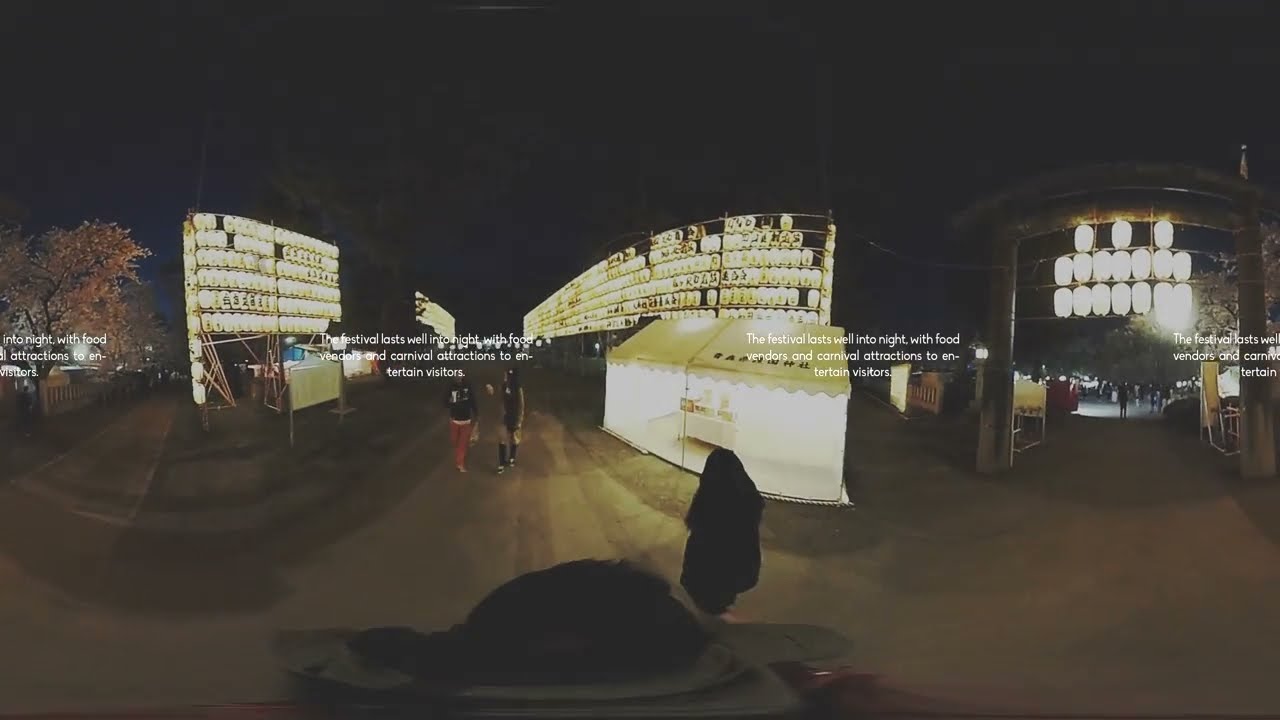The image showcases a picturesque outdoor setting featuring a curved wooden bridge with distinct knotholes and prominent red railings. Positioned centrally, the bridge spans over a small body of water and is bordered by trees with pinkish blossoms and lush green foliage. This mid-ground is complemented by a whitish light blue, slightly cloudy sky that forms the background.

The wooden deck of the bridge, visible at the bottom of the frame, has a rustic charm emphasized by its detailed texture. Surrounding the bridge, brightly colored foliage provides a scenic backdrop, with trees in bloom exhibiting vibrant pink flowers that contrast against the greenery.

The bridge is populated with numerous people walking and standing, emphasizing an active, communal environment. On the left side of the bridge, a group of about eight individuals can be seen, most donning jackets, suggesting a cool fall day. Among them, one person in a white jacket with a strap over the shoulder stands out, accompanied by individuals in a variety of outfits including black jackets, dark pants, and other mixed attire. 

On the right side, several more people are present, also dressed warmly. The people appear to be either walking or standing, enjoying the scenic view that the bridge and its surroundings offer. Overall, the image exudes a peaceful yet vibrant atmosphere, capturing both the tranquility of nature and the warmth of human presence.